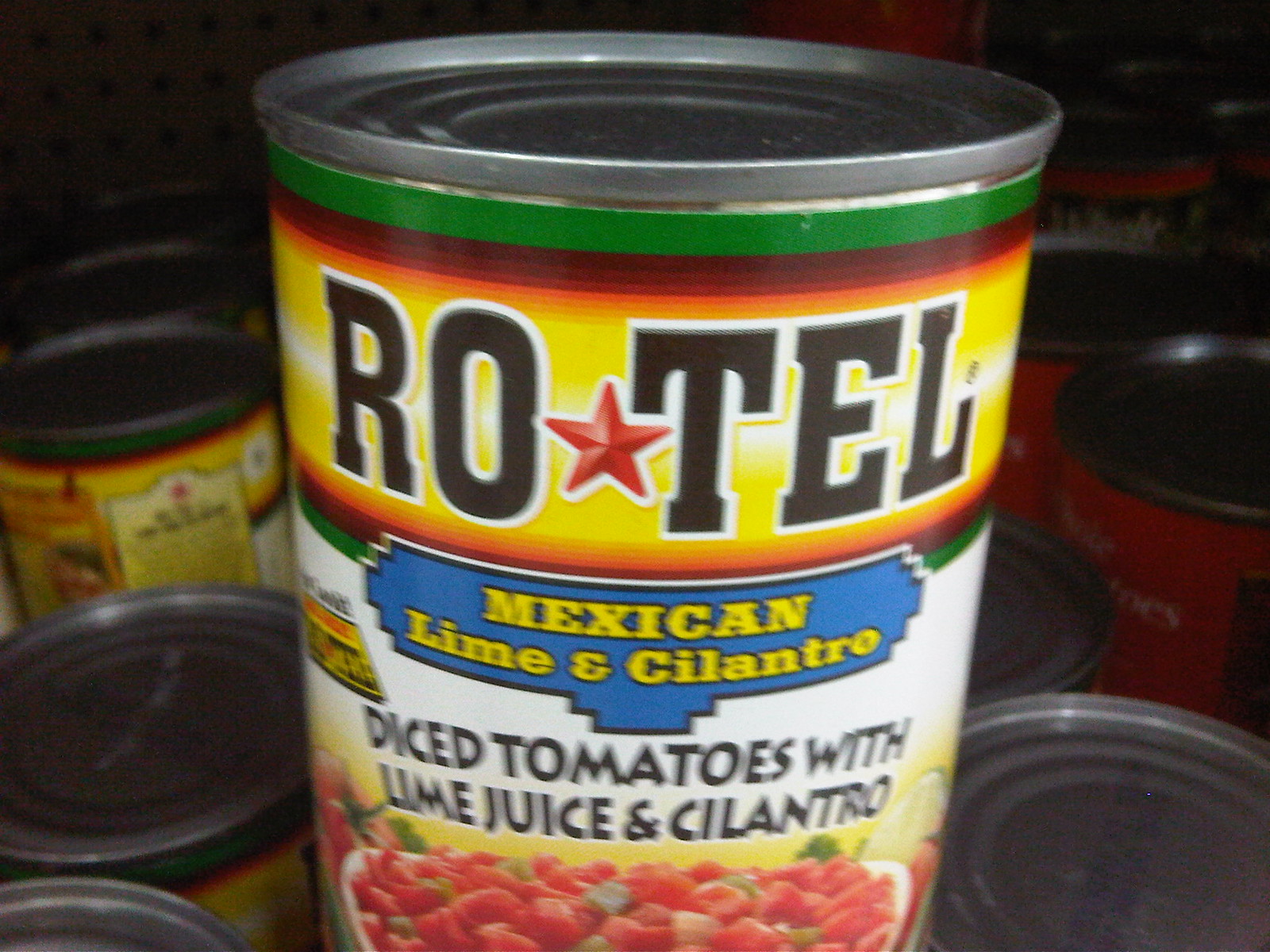This highly detailed photograph features a prominently displayed can of Rotel Mexican Lime and Cilantro Diced Tomatoes with Lime Juice and Cilantro, set in a grocery store-like setting. The can is silver and cylindrical, distinguished by its shiny surface and distinctive labeling. The label is on a white and orange background with the brand name "Rotel" in bold black text, accented by a red star between the letters. The label also features a blue badge with yellow text stating "Mexican Lime and Cilantro," and below that, in black capital letters, "Diced Tomatoes with Lime Juice and Cilantro." At the bottom of the label is a graphic showing red, cube-shaped diced tomatoes, suggesting a salsa-like appearance. In the foreground, there's a visually appealing bowl of diced tomatoes, lime juice, and cilantro, reinforcing the can's contents. The background reveals rows of other silver, cylindrical cans, as well as some orange or red-colored cans off to the right, adding depth and context to the grocery display.